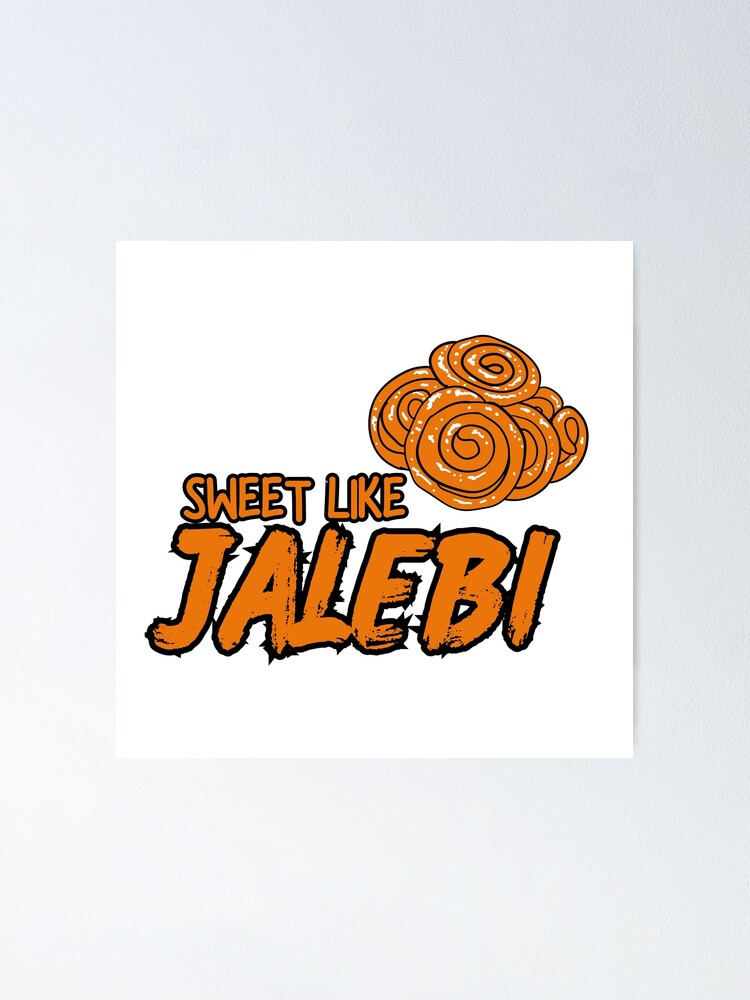The image is a detailed color illustration and logo design. The overall format is a vertical rectangle with a light gray background. Inset into the center of this gray background is a smaller white square, which contains the main elements of the illustration. On the top right portion of this white square, there's a pile of spiral-shaped discs resembling sweet rolls or cinnamon buns. These rolls are brown with an orange tint and are detailed with white speckled highlights, possibly resembling sugar or frosting. Below this pile, centrally positioned in the bottom half of the white square, the text "SWEET LIKE JALEBI" is prominently displayed in all capital letters. This text is orange, outlined in black, with a spiked black drop shadow, lending it a three-dimensional appearance. The design stylistically combines elements of color illustration and graphic design, creating a visually engaging business logo.